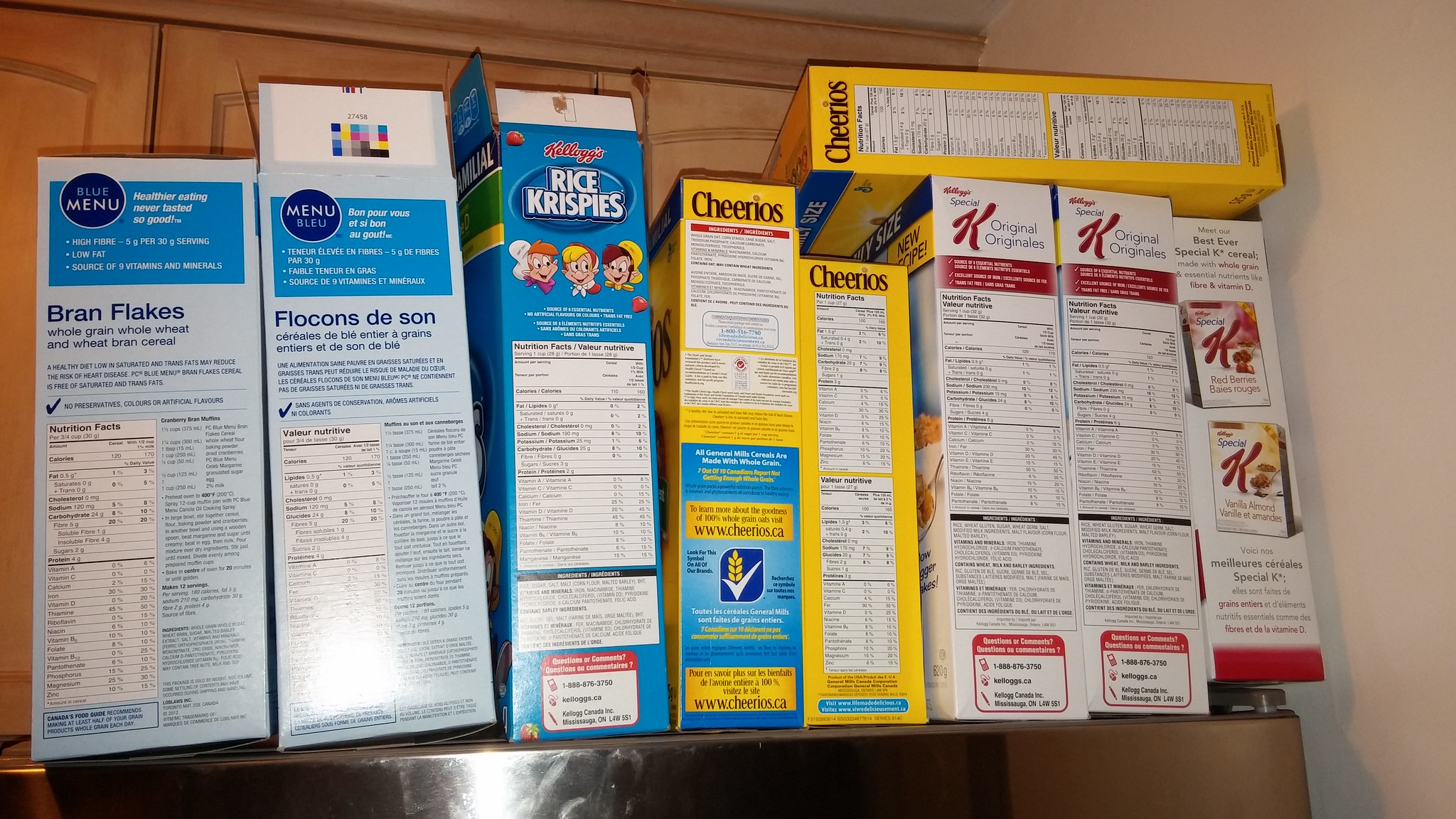This photograph captures a collection of cereal boxes neatly lined up on top of a silver metal refrigerator, set against the backdrop of brown wooden cabinets. The arrangement features nine boxes of cereal. From left to right, there are two light blue Bran Flakes boxes, each with its nutritional information visible. Next is a blue Rice Krispies box, showing the familiar three mascots—Snap, Crackle, and Pop—along with their nutrition details. To the right of the Rice Krispies are two yellow Cheerios boxes with their nutritional information displayed. Following the Cheerios are three Special K boxes; two display their nutritional facts, while the third is turned vertically. Additionally, a smaller yellow Cheerios box is placed horizontally on top of these Special K boxes. The overall presentation emphasizes the display of nutritional information on the side panels of the cereal boxes, creating a detailed and organized visual.